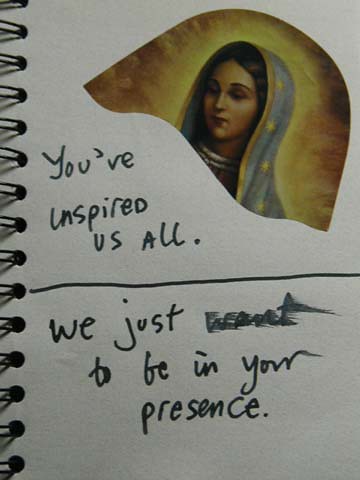In the top right corner of a dimly-lit, small notebook, spiraled on the left, an intricate cut-out of the Virgin Mary is pasted at an angle. The image depicts Mary looking downwards, wearing a blue head covering adorned with a white stripe and a yellow-gold stripe in front, embroidered with gold stars. Surrounding her head is a halo, giving off a golden aura. Below this evocative image, handwritten in black ink on the white paper, are the words "You’ve inspired us all,” underlined for emphasis. Beneath this line, it continues, "We just want to be in your presence," with the word "want" notably smudged, as if a thumb dragged the ink to the right, blurring it. The overall text, personal and raw, suggests a heartfelt tribute.